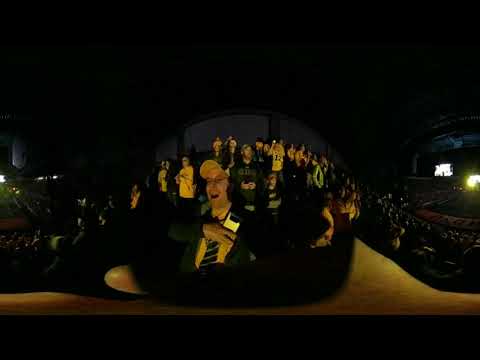The image captures an indoor nighttime scene, likely taken with a wide-angle or fishbowl lens, giving it a curved, distorted effect. In the foreground, a white man with glasses and a baseball cap, who is wearing a suit and tie, stands prominently with his mouth open, looking upwards. He is holding what looks like a cell phone. Behind him, a lively crowd fills the theater, many of whom are standing up with their hands over their hearts, possibly indicating a moment of national significance such as the National Anthem. One person in the crowd is distinguishably wearing a shirt with the number 12, and there is a man in a black hat next to a child, both looking upward. A woman in white and a person holding a lit cell phone add to the dynamic scene. The top right corner of the image features a television screen or monitor with some white writing, though it is not legible. The setting is dark, with ambient stadium lights providing minimal illumination, framing the excited expressions of the fans who appear to be thoroughly engaged in what seems to be a concert or a football game, perhaps even an Iowa Hawkeyes event, given the possible black and yellow colors observed. The crowd's thrilled demeanor and the vast, encompassing stadium suggest they are having an exhilarating time.